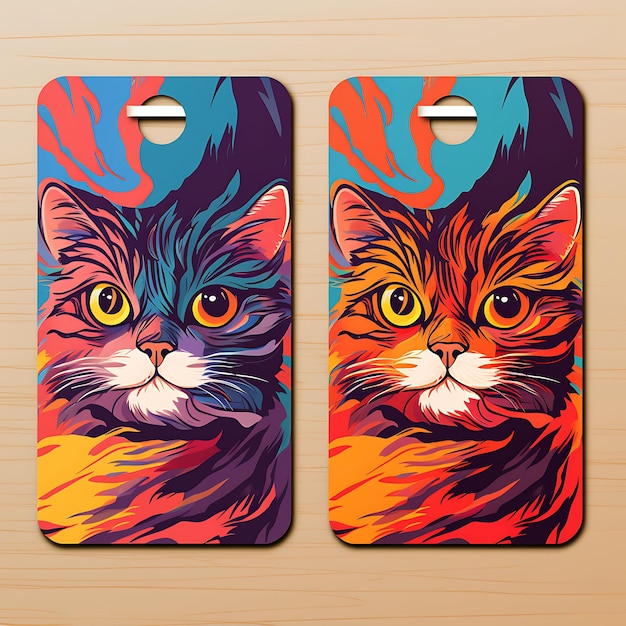Displayed against a light brown wooden surface with horizontal striations, this image features two vertically oriented phone cases hanging from a metal peg. The focal point of each case is a vibrant and colorful depiction of a cat. The phone case on the left showcases a cat with shades of pink, blue, and purple on its head, transitioning to a body infused with hues of purple, yellow, and pink. The background of this case is coral with accents of blue and purple, while the cat’s eyes are strikingly mismatched - one yellow and the other orange. In contrast, the phone case on the right presents the same cat with a predominantly orange palette, incorporating orange on its face and body accented by touches of pink, deep purple, and blue. The background here shifts to a vibrant orange and turquoise. Both cases are depicted with bold, expressive strokes, highlighting the unique artistic interpretation of the same feline subject. The image is clear and well-lit, showcasing the vivid and dynamic colors of the phone cases in sharp detail.